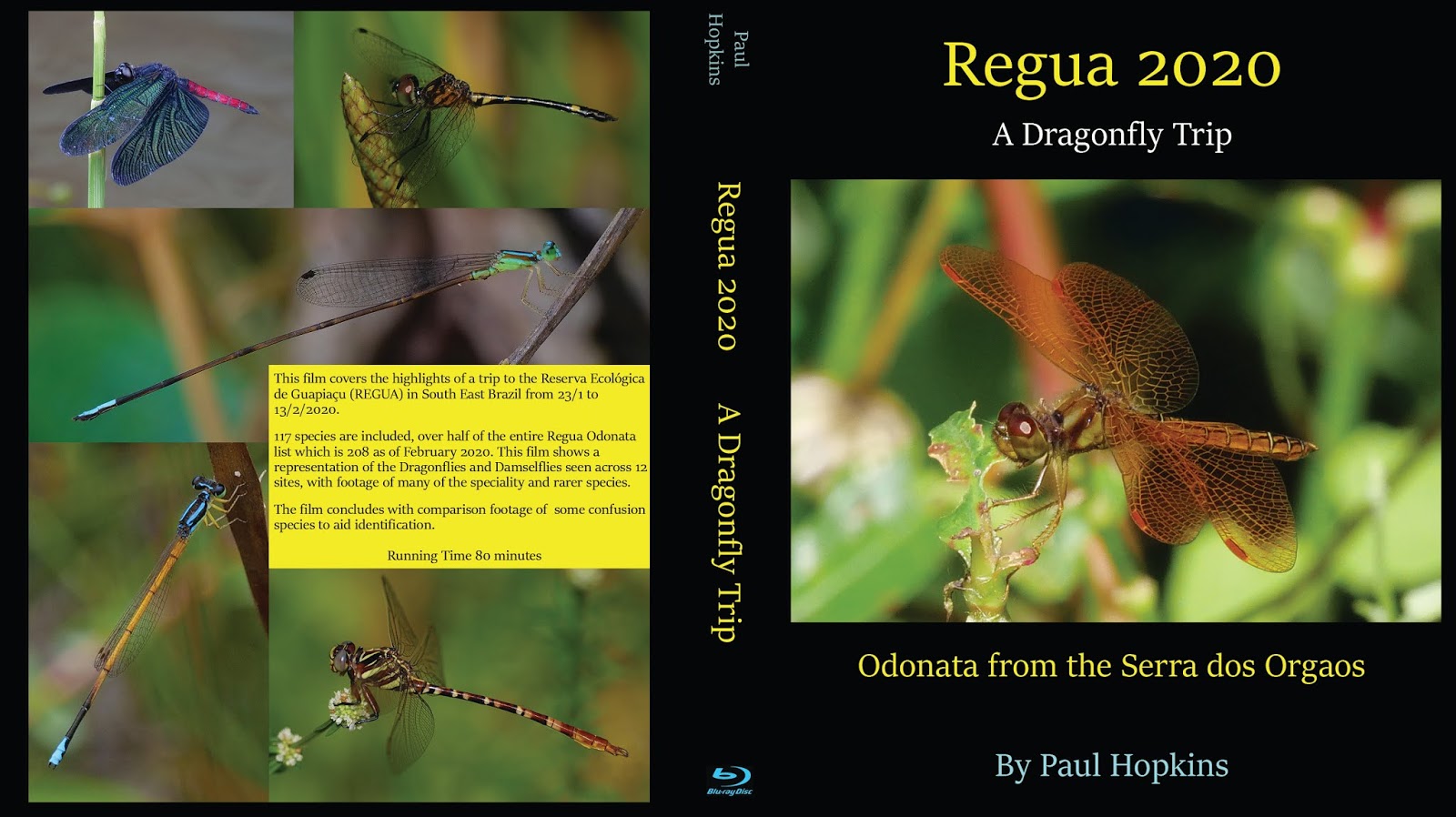A detailed Blu-ray disc cover illustration that highlights the film "Dragonfly Trip," directed by Wu-Gi-Yeh in 2020. The cover features an array of dragonfly-themed photographs and important details. On the right-hand side, there is a prominent image of a dragonfly feeding on nectar from a flower, accompanied by the text "Odonta from the Sierra Dos Orgios by Paul Hopkins." Above this, the title "Dragonfly Trip" is boldly displayed.

On the left-hand side, additional images of various dragonflies are arranged around a descriptive blurb. This text provides an overview of the film, which documents an expedition to the Reserva Ecológica de Quepico in Southeast Brazil, capturing stunning visuals and research notes from January 23 to February 13, 2022.

At the center of the cover, a larger block of text clarifies that this Blu-ray disc cover is indeed the highlight of the dragonfly exploration trip, and emphasizes the rich biodiversity and unique behaviors of dragonflies depicted in the movie. The detailed imagery and comprehensive text make it clear that this film is a vibrant and informative journey into the world of dragonflies.